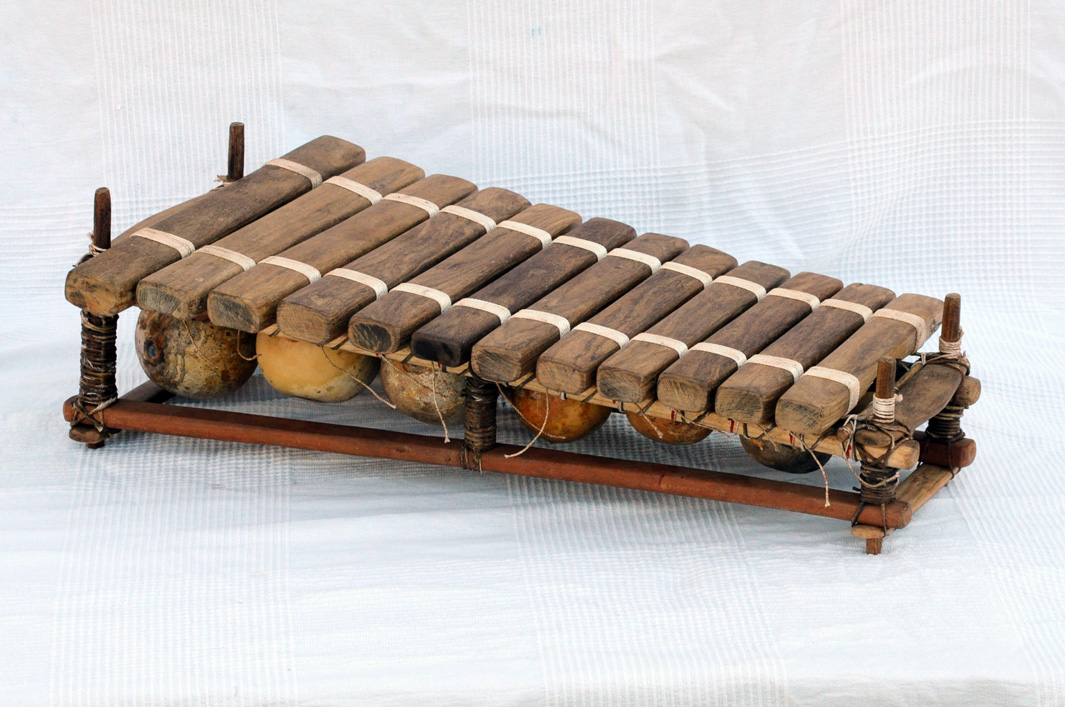The image features a handmade wooden contraption that resembles a xylophone, displayed against a white, wavy and partially checkered background. The structure consists of 12 carved wooden bars that become progressively shorter from left to right. These bars exhibit a variety of brown shades, ranging from light to dark, and show the natural grain of the wood. Each bar is secured at both ends by white bands or straps, and they are arranged side by side. The entire setup rests on a series of roughly six spherical objects, possibly made of stone or carved wood, which are situated beneath the wooden bars. These spheres display colors including light brown and grayish tones, contributing to an old, rustic appearance. Additionally, the wooden bars are anchored by vertical posts on each end, connected to a larger, dark wooden post bound with rope-like threads at the base, giving the ensemble a tribal or primeval look. The overall impression is of an instrument or a ceremonial artifact.